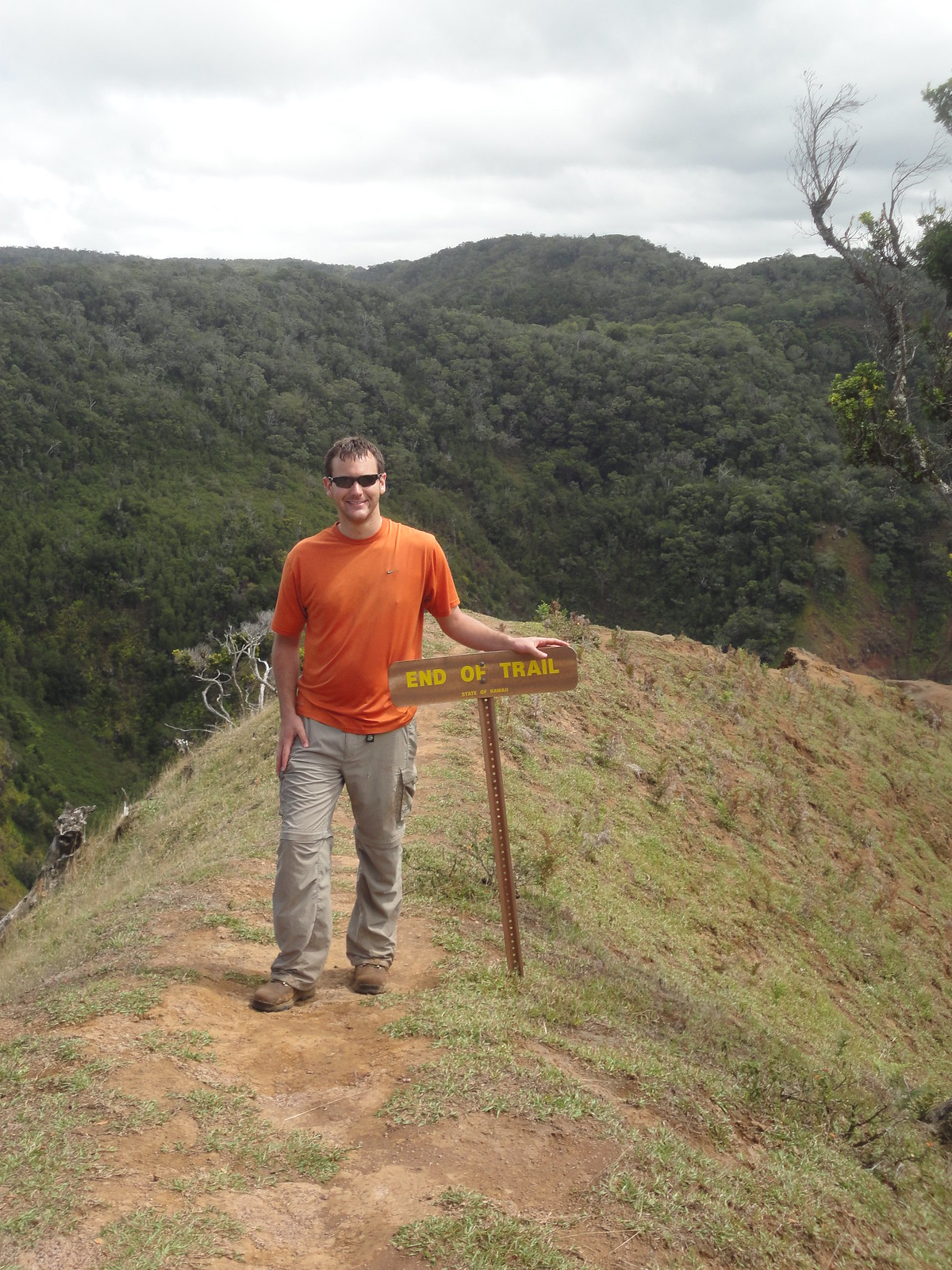In this image, we see a man standing directly in the center, leaning on a wooden sign that reads "End of Trail" in yellow letters. The man appears to be white and roughly 25-26 years old, sporting brown hair, sunglasses, an orange short-sleeved t-shirt, grayish cargo pants, and brown hiking boots. He is smiling for the photograph. He stands on a mound or hill where the ground surface is a mix of light green grass and exposed soil. 

In the background, a series of hills and mountains are densely covered with dark green trees and foliage, while the sky above is filled with white and gray clouds, indicating a cloudy day. The setting is clearly outdoors, on a hiking trail, and the mood suggests a sense of completion or accomplishment, as the man reaches the trail's end. The range of colors in the image includes various shades of green, light brown, tan, orange, yellow, white, and gray, adding to the natural and tranquil ambiance of the scene.